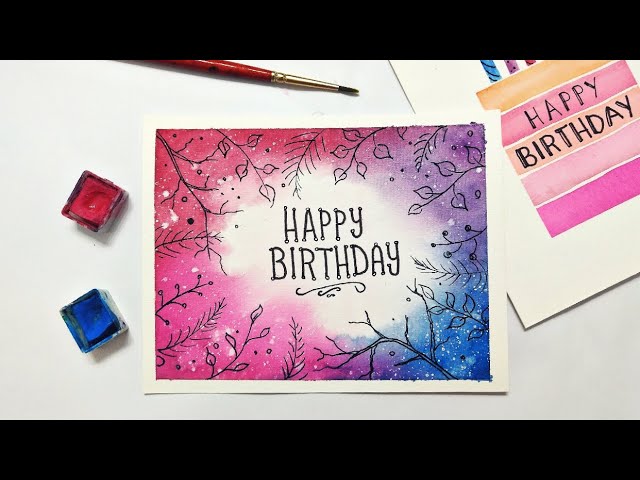In this image, we see two handcrafted birthday cards prominently displayed. The primary card in the center of the image features a "Happy Birthday" message with an artistic design of black-outlined trees and plants surrounding the text. Above this central card, a brown paintbrush is positioned horizontally with its tip facing right. Nearby, on the left side of the card, there are two paint containers, one red and one blue, indicating the handmade nature of these cards. 

To the top right corner of the image, there is a secondary birthday card depicting a square birthday cake adorned with candles. The cake showcases a blend of pink, blue, purple, and yellow hues. Both cards exhibit meticulous artistry, emphasizing their handcrafted quality with vibrant colors and intricate designs.